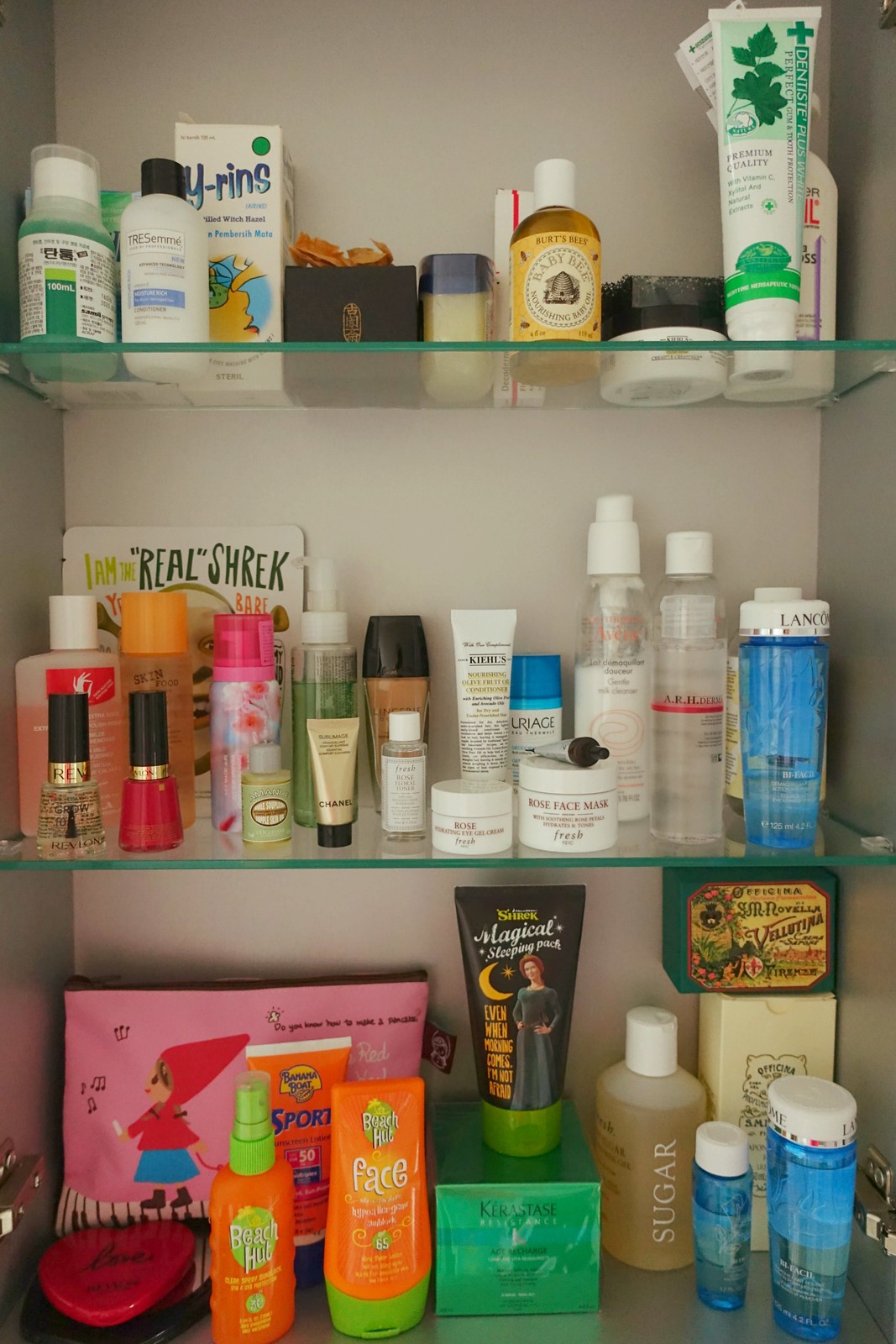This color photograph showcases a neatly organized bathroom cabinet with three shelves adorned with various personal care products. On the top shelf, we see a tube of premium quality Dentiste Plus White toothpaste, accompanied by a bottle of Burt's Bees Nourishing Baby Oil, and a Tresemme Moisture Rich product, which hints at a well-thought-out hair care routine.

The middle shelf is dedicated to an assortment of skin care items. It includes several Revlon nail polishes, a jar of Chanel cream, a bottle of Fresh Rose Toner, a Rose Face Mask, Kiehl's nourishing cream, a distinctive blue bottle from Lancome, and a few products from Avene, suggesting a focus on comprehensive skin care.

On the bottom shelf, the vibrant array of products stands out. Here, you can spot items from the Beach Hut brand, a unique Shrek Magical Sleeping Pack, a selection of Kerastase products for advanced hair therapy, several items from the Sugar brand, and additional blue bottles from Lancome, indicating a commitment to both skin and hair care.

Every item on these shelves speaks to a dedication to high-quality personal care routines and a preference for well-established, reputable brands.